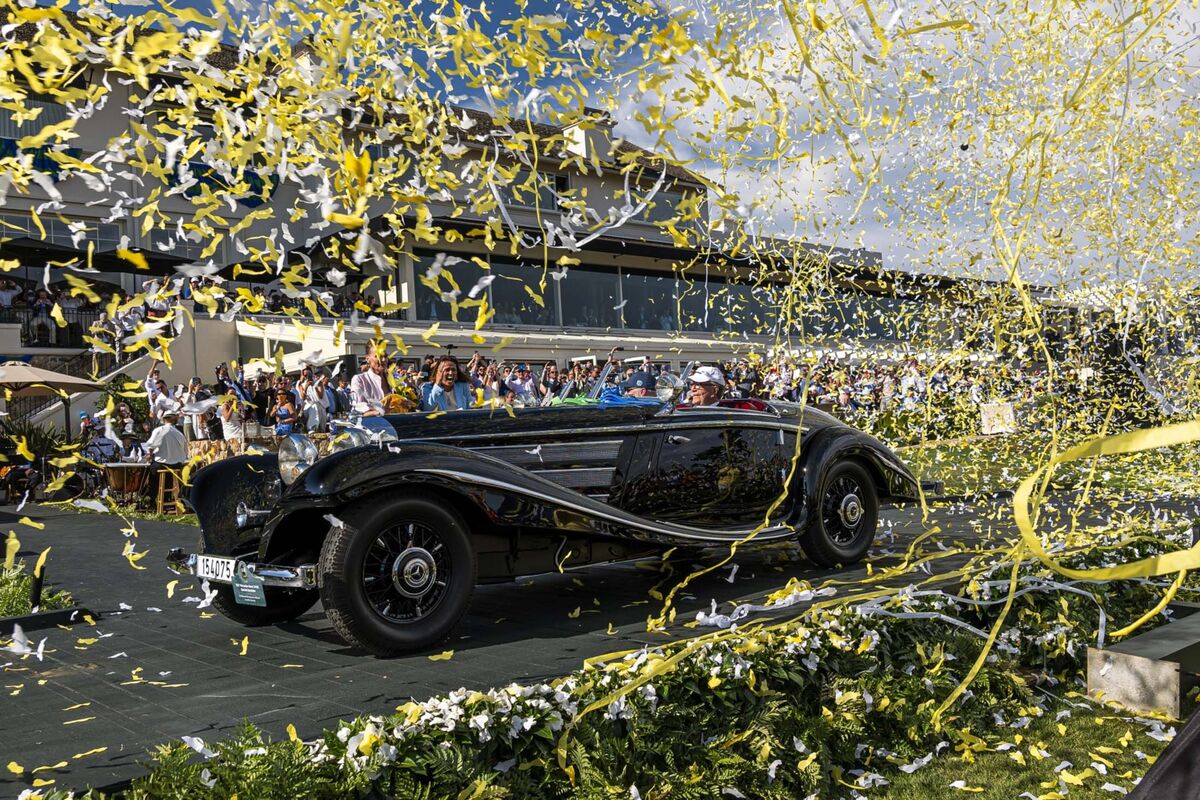This photograph captures a celebratory parade featuring a long, shiny, stylized, black Rolls Royce convertible driving through a roadway adorned with yellow and white confetti and streamers. The focus of the image is on the car, where two elderly men are seated. The man closest to the camera wears a white cap and glasses and is smiling, while the other man further back is in a blue hat. Lining the street, a well-dressed crowd is cheering, clapping, and likely celebrating a significant win, possibly hinting at a Kentucky Derby-like event with festive, ceremonial vibes. Paper confetti and streamers are festooned in the air and scattered on the ground, adding to the jubilant atmosphere surrounding the parade.